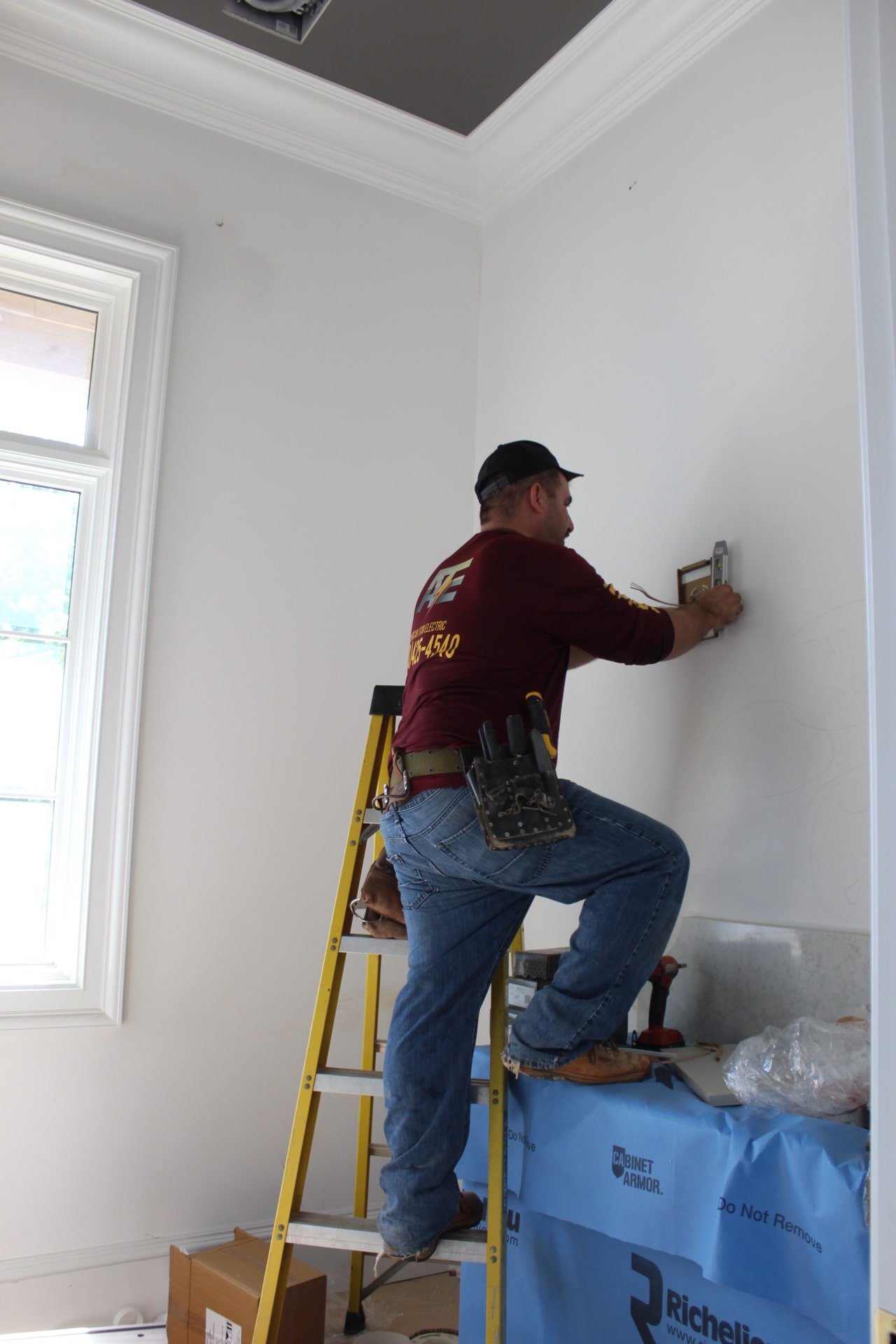A construction worker is carefully balanced on a yellow metal ladder in the midst of home maintenance work. His right foot is resting securely on a covered blue structure, likely a fireplace area temporarily shielded for protection during the renovation. Outfitted with a well-stocked tool belt, he appears to be installing an electrical hookup on a plain white wall. To his left, another wall reveals a partial view of a window. Below him, a box sits under the ladder, surrounded by various tools scattered near the blue-covered block area. The scene is a snapshot of meticulous craftsmanship amidst a home improvement project.